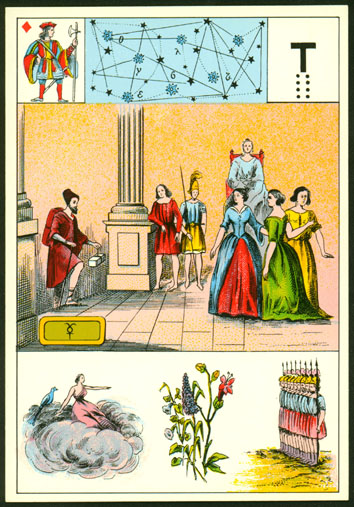This intricate and vibrant image is encased within a black frame with a white inner margin, followed by a finer, light black border. The top-right corner of the image features a figure reminiscent of a joker, identified by a prominent red diamond shape on its left side, holding an axe. The image centers around a blue and black-lined illustration, aligned with a white background featuring the letter 'T' in black, flanked by eight dots on either side.

In the central area, three elegantly dressed women are depicted: the one in the middle is clad in green, the one on the right in yellow, and the one on the left wears a blue top paired with a red skirt. To the far left, a man stands, dressed in red and holding a small package. The scene's backdrop is a yellow wall with an off-yellow column, against which a man in red leans. Adjacent to him is a soldier adorned in attire split into yellow at the bottom and light blue at the top, topped with a yellow helmet. Behind them, another man sits elevated on a red throne, clothed in light blue.

At the bottom of the composition, a line of soldiers stands on the right, positioned on brown soil. The middle ground features some plants interspersed among the visual elements. On the left, a depiction of a brown cloud cradles a woman dressed in pink, who appears to be pointing towards a blue bird with a black tail beside her. The overall composition vividly intertwines various characters and elements, creating a rich tapestry of colors, movements, and interactions.